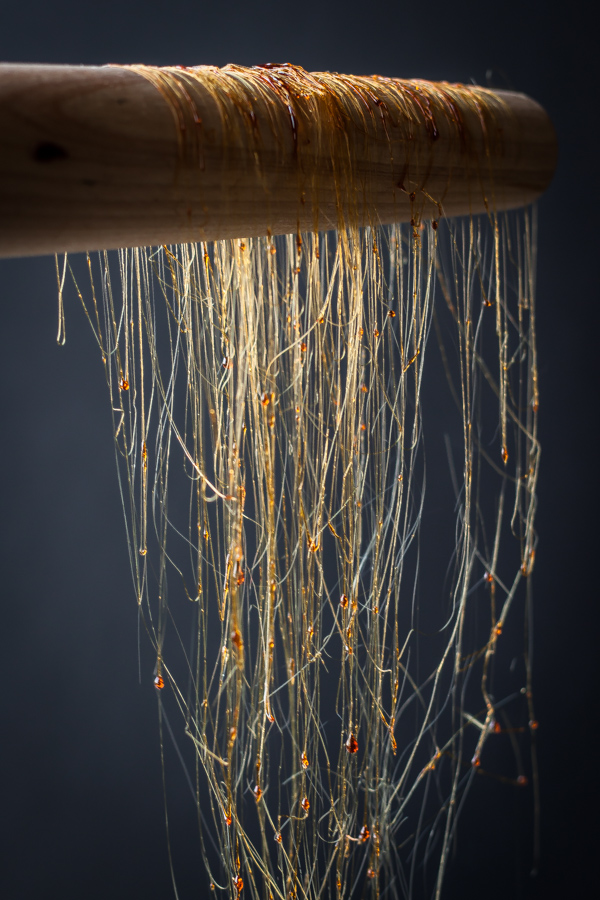The image is a vertically aligned rectangular picture featuring a prominent wooden object, resembling a rod or possibly a baseball bat, positioned diagonally from the upper left to the upper right. The wood is adorned with intricate dark grains and appears to be a medium to dark brown, with some areas around the top darker due to a coating of a sticky, amber-like substance. This substance manifests as hundreds of thin, hair-like strands hanging from the wooden rod. These strands vary; some are straight, while others are curved or ballooning out, likely where the stickiness is pooling. Certain strands are clumped together, forming thicker sections, while others remain individual. They shine golden in the light, reflecting a honey-like or caramel hue, and appear to have droplets of this amber substance scattered along their lengths. The background features a dark blue to gray gradient, making the wooden rod and its golden, sticky strands stand out sharply against the dimmer surroundings. The central part of the image is particularly well-lit, highlighting the texture and color contrast of the wood and the amber-coated strands.